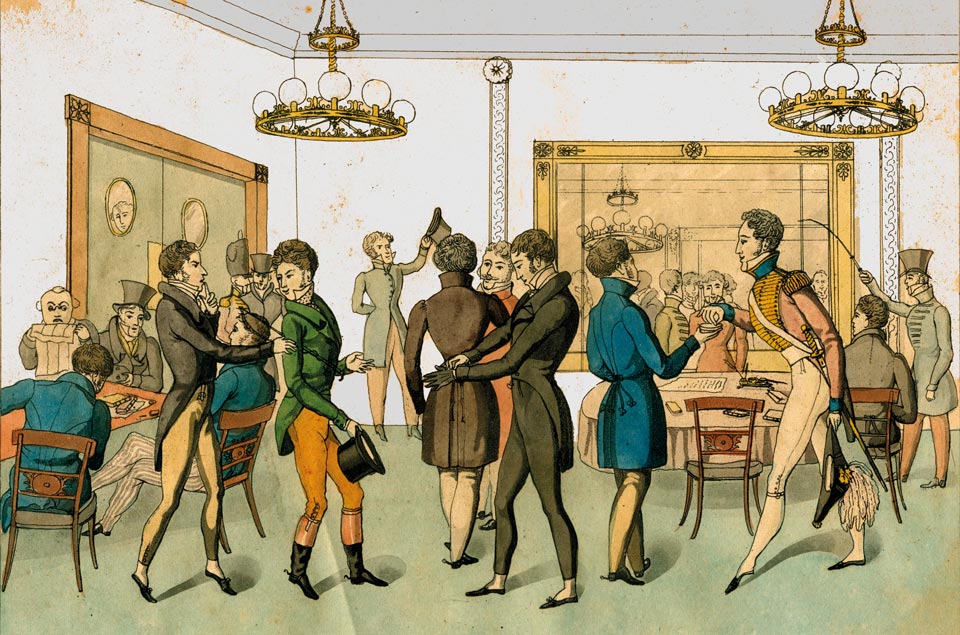The image is a detailed, illustrated color drawing set in a square room adorned with elements suggesting an 18th or 19th-century setting. The room has grayish-white walls and is furnished with wooden tables and chairs, some of which are occupied by men deeply engrossed in looking at paperwork or engaging in conversation. The men, approximately twenty in number, are dressed in period attire featuring tight-bottom pants, jackets with tails, and top hats, reminiscent of the 1700s. Notably, one figure who stands out appears to be in a French military uniform, complete with fringes on his shoulder pads and a feathered hat, indicating high status.

The background features a large mirror or picture dominating the wall and reflecting parts of the room, creating an illusion of depth. There are two double swinging doors on the left wall, each with round windows at the top; one of these windows frames a man peering through. Adding to the room's elegance, two gold chandeliers hang from the ceiling, their round metal frames adorned with globes encircling them. The scene is lively, with men scattered around the room, some standing and talking in the foreground, while others sit and interact more subtly in the background. One man is even seen tipping his hat, capturing a moment of social engagement in this richly detailed tableau.